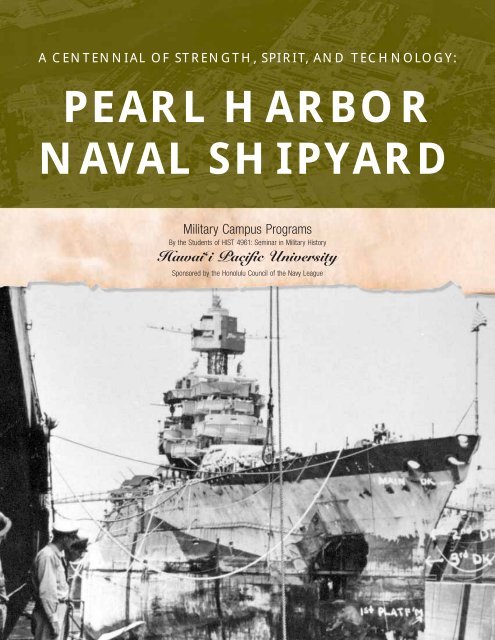The image is a detailed announcement for an event or program related to military history. At the top of the image is an olive green rectangle with the title "Centennial Strength, Spirit, and Technology" written in white, followed by "Pearl Harbor Naval Shipyard" in a larger font. Below this is a cream-colored piece of paper, seemingly torn at the bottom, which reads "Military Campus Programs" in black. The finer print below includes "by the students of SHG 4961 Seminar in Military History, Hawaii Pacific University," sponsored by "Honolulu Council of the Naval League." The lower half of the image showcases an old black and white photograph of a large battleship docking or coming into dock. This ship is seen up close with two uniformed naval personnel standing to the right, possibly interacting with the ship or managing docking ties. The photograph provides a nostalgic glimpse of the maritime history associated with Pearl Harbor.